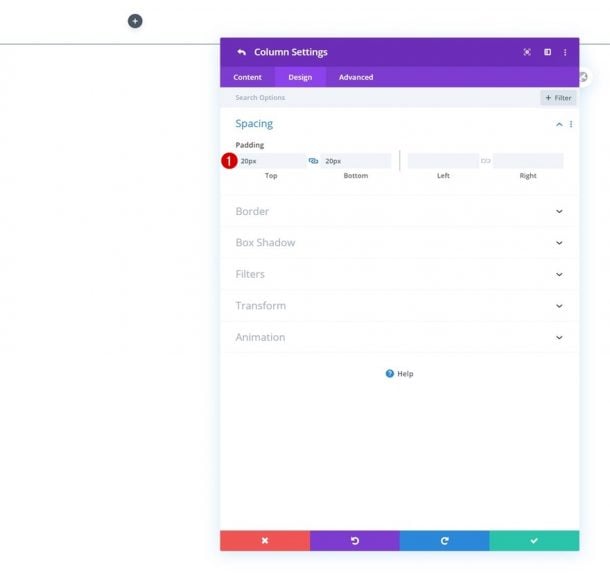This is a detailed screenshot of a user interface with a white background, showcasing various customization and navigation elements. At the center, there is a prominent gray circle featuring a white plus symbol. To the top-left, a back arrow is visible, allowing users to navigate to previous menus. The screen displays several sections, including 'Content', 'Design', 'Advanced Search Options', and 'Filter'. The 'Filter' section is highlighted with a gray rectangle containing black text and a black plus symbol. 

Adjustable design parameters like 'Spacing' and 'Padding' are noted, with an example showing red circles containing the number '1' next to '20px' for both top and bottom padding. There are also gray rectangles labeled 'Left' and 'Right', likely representing alignment settings. Each section has down arrows indicating expandable options, such as 'Border', 'Box Shadow', 'Filters', 'Transform', and 'Animation'.

Additionally, a blue circle with a white question mark marked 'Help' is present for user assistance. At the bottom of the interface, there are functional buttons including an 'X' to close, 'Undo', 'Redo', and a 'Check Mark' for confirming changes, each housed in uniquely colored rectangles for easy identification.